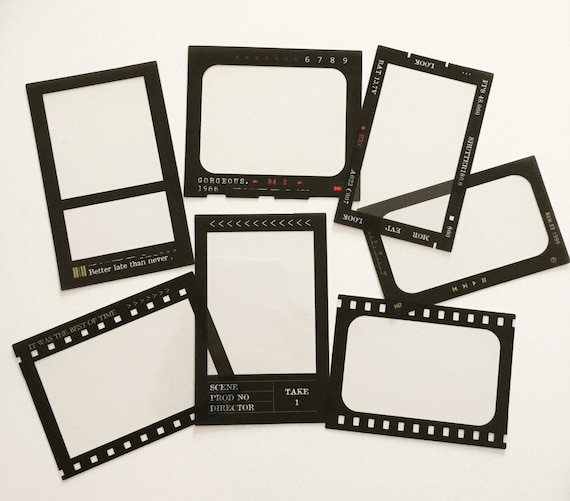The image displays an assortment of black-framed items and holo analog films scattered on a light grey or white surface. These various black-bordered frames and posters are adorned with motivational texts and potential movie-related phrases. Prominent texts include "gorgeous 1988," "better late than never," and "it was the best of times." One particular frame, resembling a clapperboard used in filmmaking, features labels like "scene," "prod number," "director," and "take 1," with the inside frame left blank. Other smaller texts such as "look" and "eat" are also visible but are harder to decipher. The overall arrangement suggests a thematic blend of motivational saying and cinematic elements.